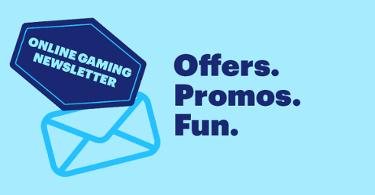Here is a refined and detailed caption based on the provided description:

"The image is a small, rectangular online flyer or banner for an online gaming newsletter. The background is a light blue hue, creating a visually appealing contrast with the darker blue text. Positioned on the left side of the banner is an icon representing an envelope, symbolizing newsletter communication. Above the envelope, a stylish banner prominently displays the text, 'Online Gaming Newsletter,' indicating the purpose of the communication. Adjacent to this, it reads, 'Offers, Promos, and Funds,' suggesting that the newsletter will contain valuable content related to special deals and financial opportunities in online gaming. The overall dimensions of the image are compact, akin to the size and shape of a credit card, making it easily viewable and shareable. This banner image effectively serves as an inviting introduction to an online gaming newsletter, without providing additional details."